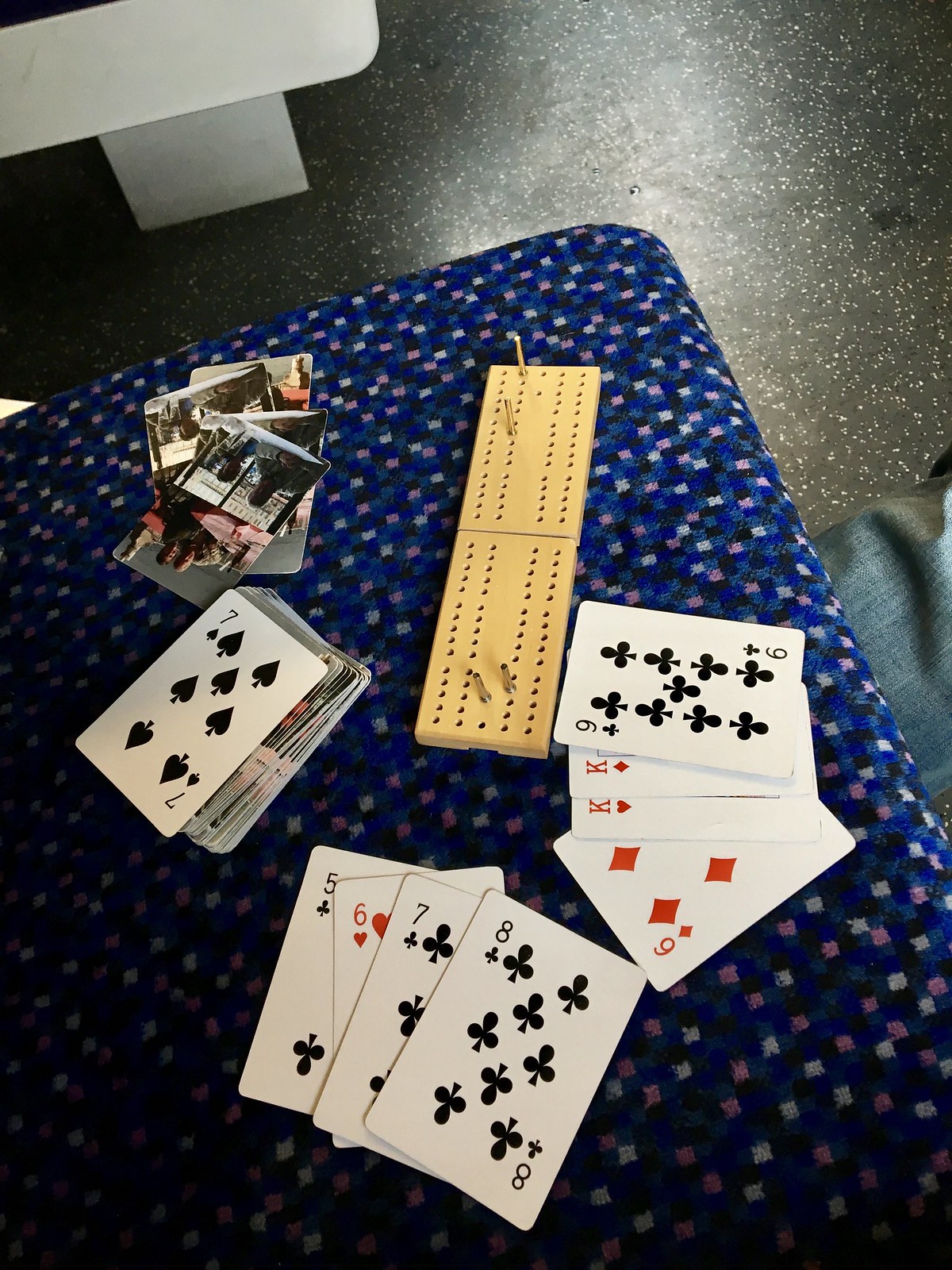In this image, a variety of playing cards are scattered on a floor with a cushion nearby. The cushion features a checkered pattern with dark blue, black, and white squares. Among the cards, a few are displayed in a hand-like arrangement with a sequence showing a 5, 6, 7, and 8 of various suits. Additionally, there is a cluster that includes a 6, two Kings (one of hearts and one of diamonds), a 9 of clubs, an 8 of clubs, a 7 of clubs, a 6 of hearts, and a 5 of clubs. On top of a neatly stacked deck, a 7 of hearts card is prominently placed. Among the cards are a few with illustrations of people. Beside the cards, two wooden squares with holes on the left and right sides, bearing metal pieces vertically aligned on each side, can be seen. The floor in the background has a black surface speckled with white. Partially visible in the right side of the image is a denim-clad leg, and a whitish, indistinct object is also present in the background.